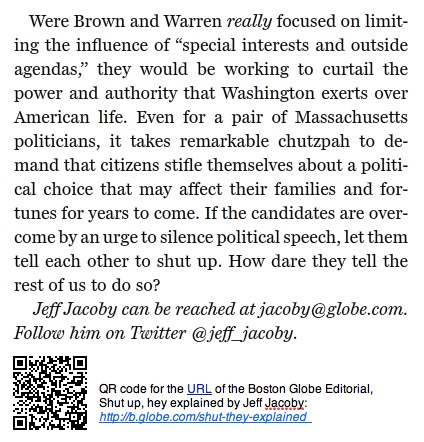Here is the cleaned-up and detailed caption for the image:

---

The image features an excerpt of text from an editorial by Jeff Jacobi, prominently discussing the topic of political speech and influence in America. The article critically examines the actions of Massachusetts politicians, Brown and Warren, arguing that their focus should be on reducing the power and authority wielded by Washington over the lives of American citizens. The text suggests that it is audacious for these politicians to expect citizens to remain silent about political choices that significantly impact their lives and futures. Jacobi goes on to assert that if the candidates wish to suppress political speech, they should direct that sentiment toward each other rather than towards the public. 

In the bottom left corner of the image, there is a QR code leading to the full editorial titled "Shut Up, Explained" by Jeff Jacobi, published in the Boston Globe. The text provides the URL (http://b.globe.com/shut-they-explained) for direct access and includes Jeff Jacobi's contact information (jacobi@globe.com) and his Twitter handle (@Jeff_Jacobi).

---